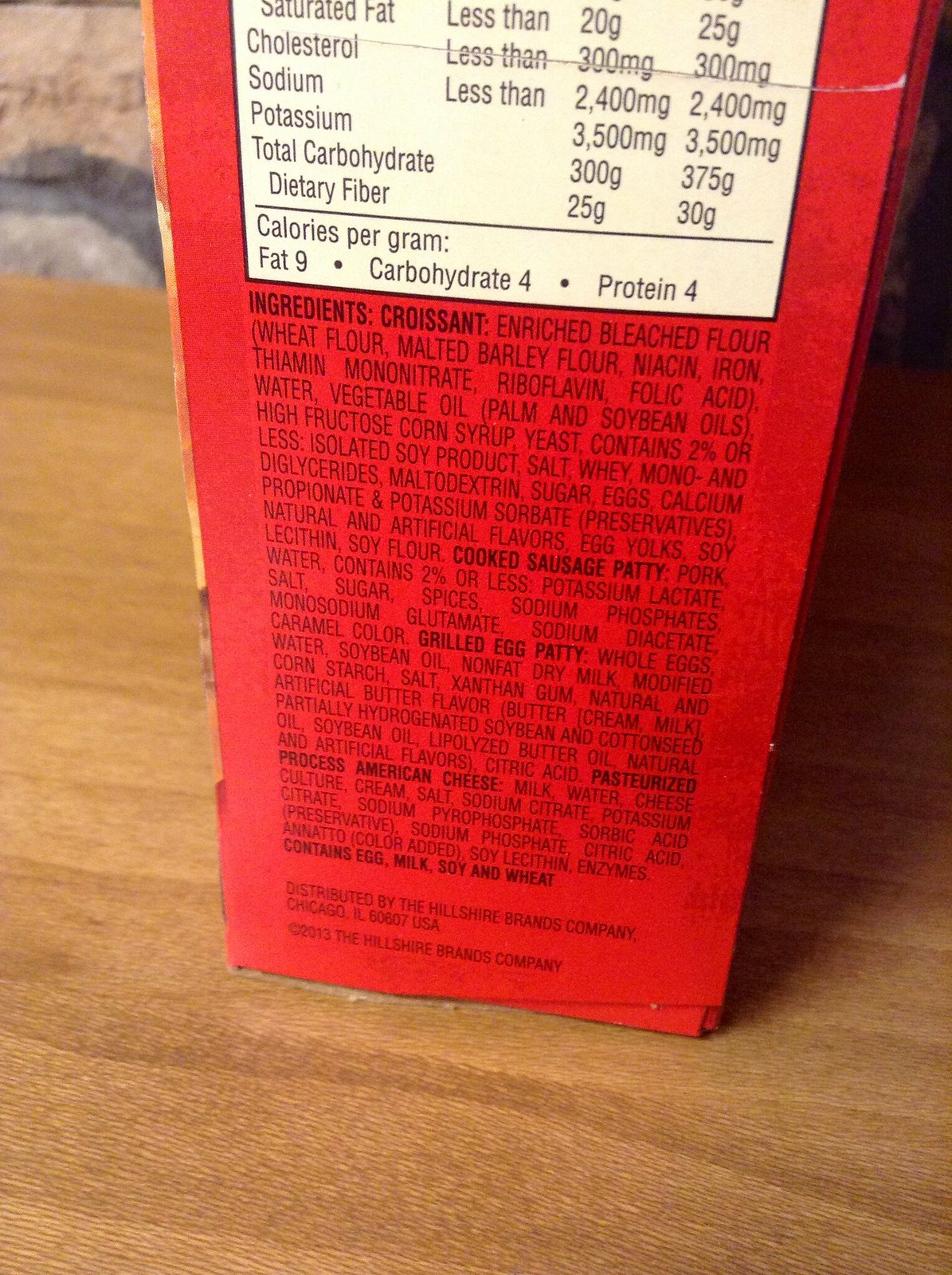This is a detailed photograph showcasing the lower portion of the side panel of a food product box, which is primarily red in color. The box, identified as part of the Hillshire Brands Company from Chicago, Illinois, dated 2013, prominently sits on a wooden surface, with a stone wall serving as the backdrop. The packaging suggests it contains croissant sandwiches filled with a combination of sausage, egg, and cheese. The visible part of the box features a split section: the upper part includes an ivory-colored rectangle with writing, while below that, black text contrasts against the red background listing nutritional information such as saturated fat, cholesterol, sodium, potassium, and total carbohydrates, which is noted to be 300 grams. Moving further down, the ingredients are outlined in detail, starting with the croissant made from enriched bleached flour (wheat flour, malted barley flour, niacin, iron, thiamine mononitrate, riboflavin, folic acid) and other components including vegetable oil and high fructose corn syrup. The cooked sausage patty's primary ingredient is pork, followed by the grilled egg patty and pasteurized processed American cheese, where milk is the primary component. Additionally, the packaging displays dietary content like calories per gram, emphasizing the comprehensive ingredient list and nutritional data for the product.